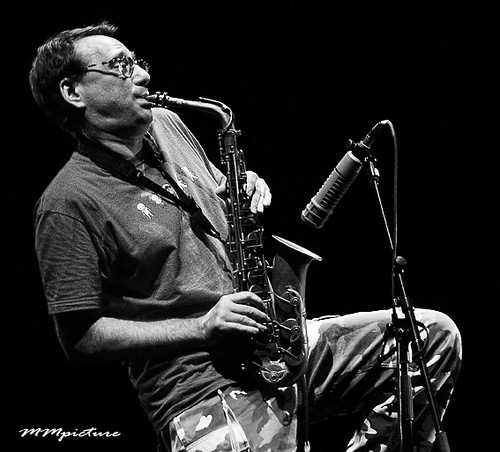The black and white photo captures a man seated on a stool playing a saxophone, held by a strap around his shoulder. He is dressed in khaki pants and a black t-shirt with some writing on the front, with slightly wrinkled sleeves. The man has short, black hair and glasses. One leg is raised while the other rests down. In front of him, a microphone on a stand points downwards towards the saxophone's end. The background of the image is entirely black, and at the bottom of the photo, there is white text that reads "MN Picture."